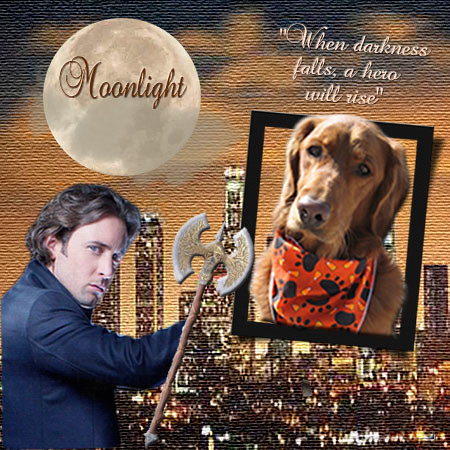The image is a well-composed graphic design that combines color photography, illustration, and typography in a square format, resembling the front cover of a movie or a book. In the bottom left corner, there is a photograph of a man with a lighter skin complexion, dark hair, and a dark suit, looking over his right shoulder. He is seen holding a medieval-style axe. Above him, in the top left corner, there is an image of the moon with the word "Moonlight" overlaid in beige script lettering. The right side of the image features a brown dog wearing an orange scarf adorned with black and yellow paw prints. The dog's head is partially framed in black, and just above, text reads, "When darkness falls, a hero will rise." The background is dominated by an aerial photo of a city skyline at night, with illuminated buildings and skyscrapers. The overall scene is set outdoors at night, filled with colors including black, grey, tan, brown, orange, and yellow, all well-spaced and easy to see. The style merges photographic realism with graphic design elements to create a dramatic and cohesive visual narrative.